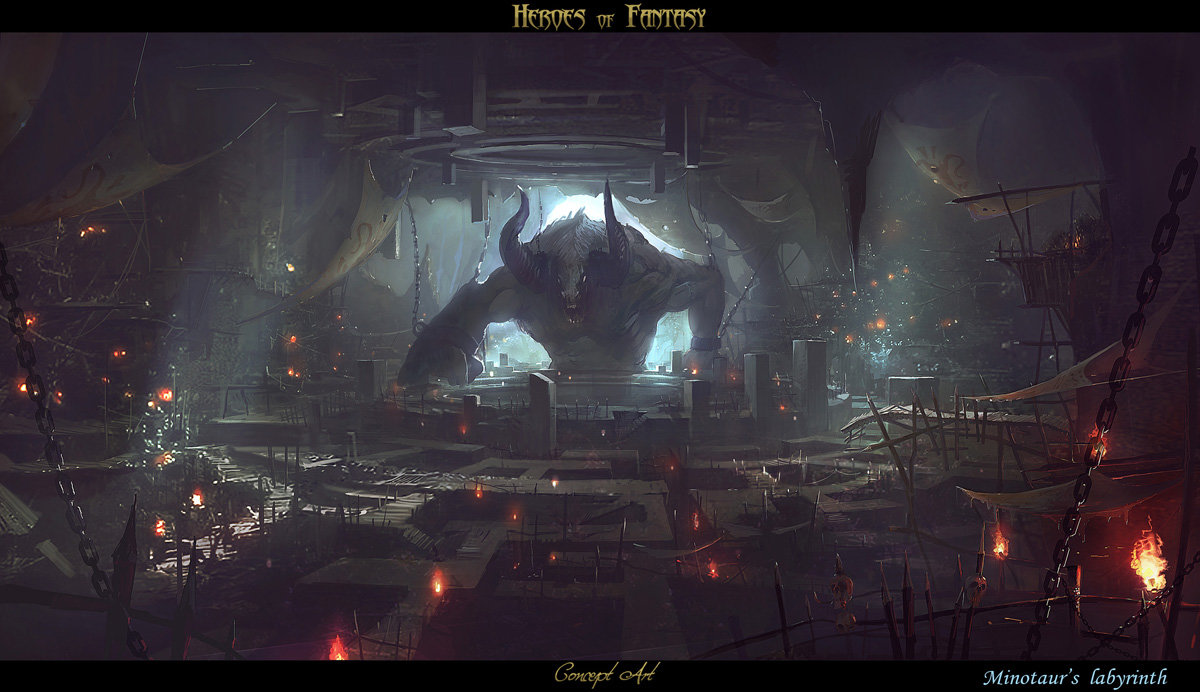The image appears to be a screenshot from a video game titled "Heroes of Fantasy," prominently displayed in white text at the top of the image. The scene is set within a dark, cave-like chamber illuminated by multiple fire lamps, chains, and various other elements that contribute to its foreboding atmosphere. Central to the image is a massive Minotaur, identifiable by its large horns, emerging through a brightly lit entrance. The colors are predominantly dark, with shades of black, brown, and gray dominating the background, while vibrant hues of orange, yellow, and red highlight the fire elements. At the bottom of the image, the text "Minotaur's Labyrinth" is visible, suggesting the setting within the game. The overall theme is dark and fantastical, with intricate details that create an immersive and intense environment.